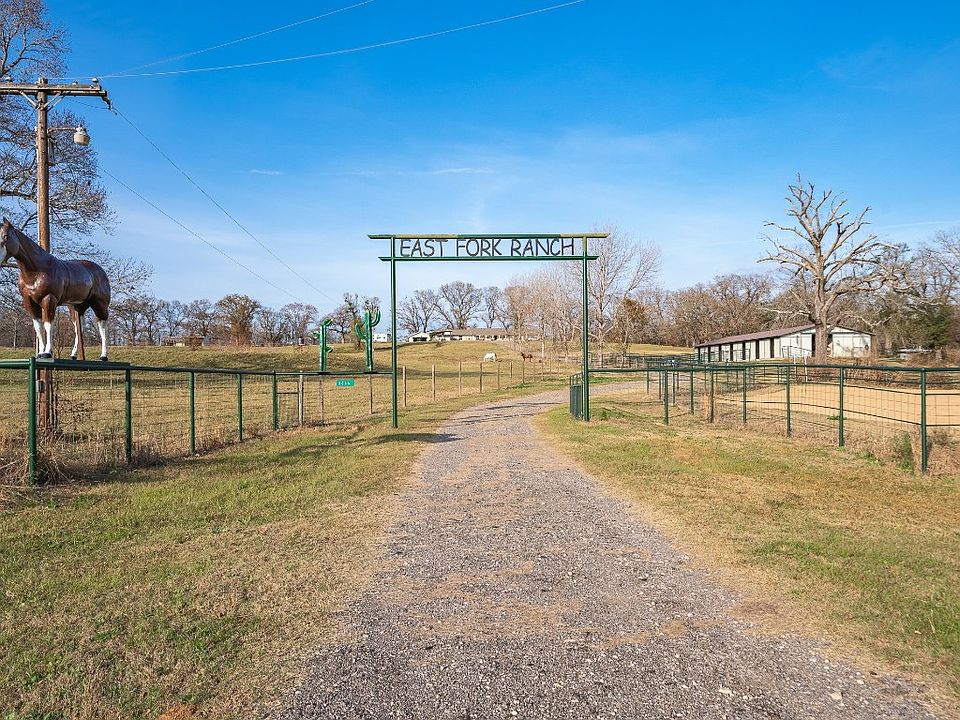The image showcases the entrance to East Fork Ranch, marked by an archway sign with large green text standing on green posts. A gravel road runs straight down the middle, framed by green fences on either side with grassy margins. Atop one of the fence posts on the left, there's a statue of a brown horse with white legs and black hooves. In the distance, faint outlines of real horses are visible. To the right of the road, a leafless tree stands in front of a white stable with a dark red roof. The clear blue sky is dotted with light clouds, and power lines can be seen in the background. The scene is captured on a sunny day, providing a welcoming view of the rural ranch.